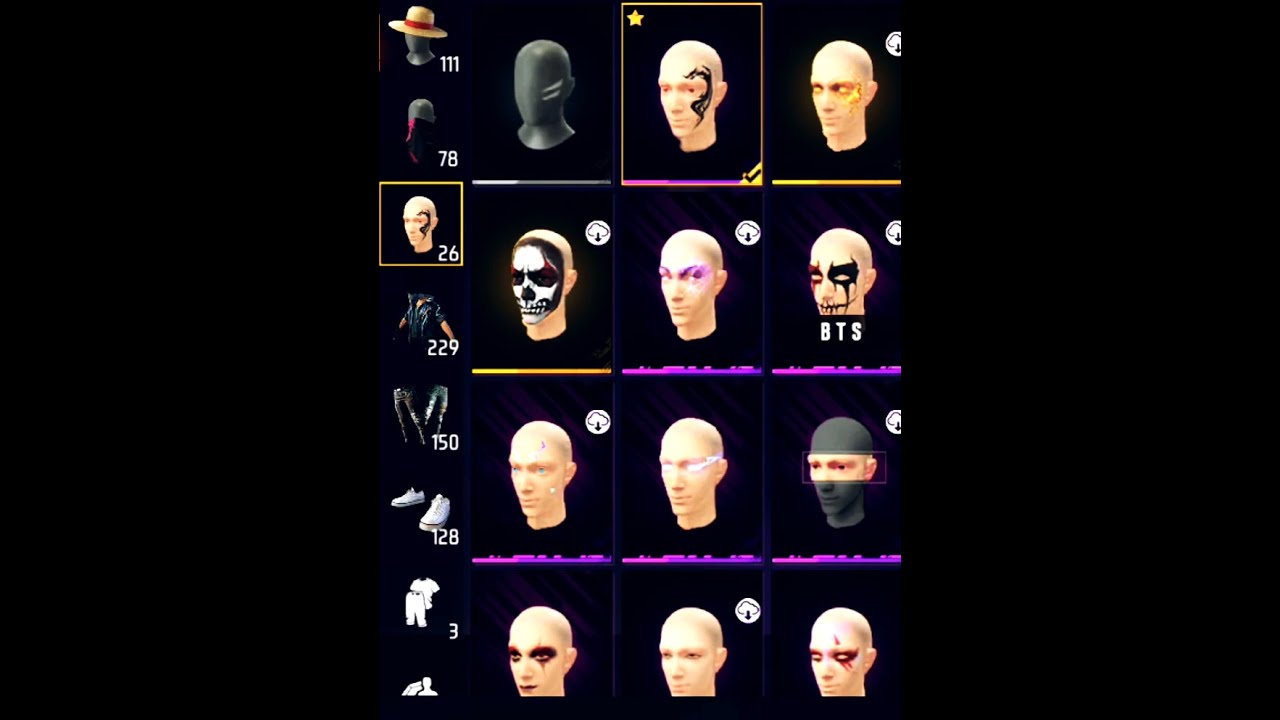The screenshot from the video game showcases an extensive character customization menu focused on facial makeup and cosmetic treatments for the character. Dominating the central portion of the screen is an avatar displaying various facial designs, with the currently selected option marked by a yellow outline and a star. This selection, itemized as choice number 26, features a dragon tattoo embellishing the avatar's face. The side panels offer a comprehensive selection of customizable elements, including hats, face masks, tattoos, jackets, pants, boots, and tops.

The left section contains four distinctive categories and their subsequent options, organized into three columns and four rows. Among these options are a fully black mask, a white face with a dragon tattoo, a face with red eyes suggesting a possessed appearance, a skull face, and other faces adorned with various makeup designs, such as dark eyeliner, purple makeup, and detailed paint schemes. Noteworthy selections include faces with horns, intricate eyeliner patterns forming tears, scars, and more. The customization menu allows for a high degree of personalization, giving players the option to craft unique and expressive avatars.